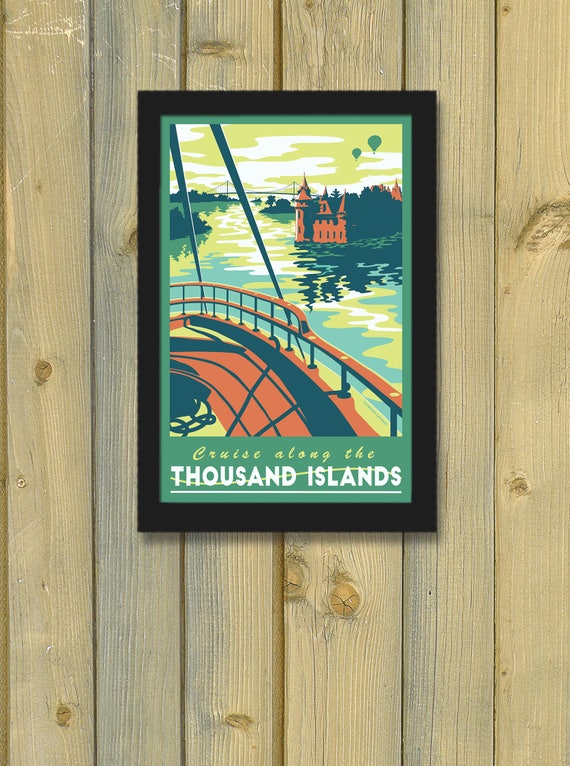The image features a vertical rectangular picture hanging on a light-colored wooden wall with vertical planks. The picture is framed in black, with an inner green border that lines the artwork. The artwork depicts a scene from a boat, identifiable by its railing in the lower part of the image, rendered in pastel reds and browns. The scene includes a body of water extending into the distance towards the upper left, flanked by green areas on both sides. To the right, there's a large castle-like building in orange. The water is depicted in shades of blue, green, and yellow, creating wavy patterns. The sky above has a yellow tint with white clouds. Two green balloons are visible in the upper right corner. Two lines descend from the upper left towards the bottom frame, suggesting boat rigging. Below the artwork, text in small yellow writing reads "cruise along the," and beneath that, in larger white writing, it says "thousand islands," which is underlined.